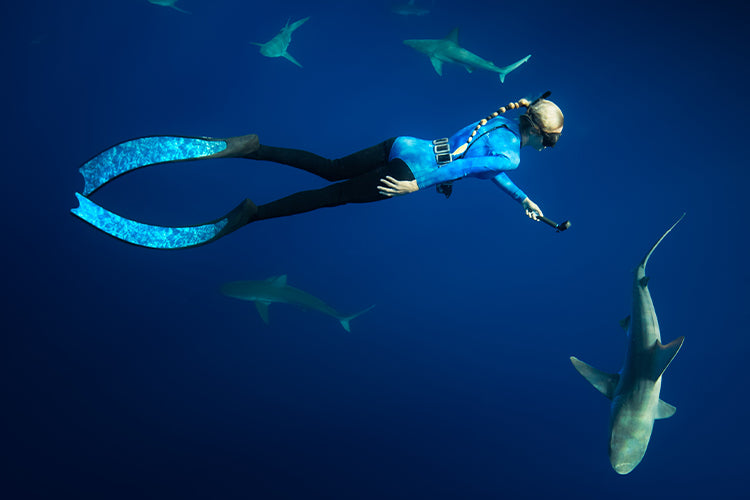In this stunning underwater photograph, a sleek shark adorned with radiant yellow-golden circles swims gracefully through the sapphire blue ocean. The light from these bright circular patterns illuminates its skin, defying the darkening edges of the water. Close by, a woman diver with long, braided blonde hair stretches out in a swimmer's pose. She mirrors the shark's elegance, her wetsuit mimicking the shark's intricate circular patterns. Equipped with exceptionally long fins, she swims just inches away from the shark, creating a harmonious scene. Despite their proximity, the shark remains unperturbed by her presence. The tranquil, still water encapsulates the duo, with the surface and its reflective shimmer faintly visible above them.